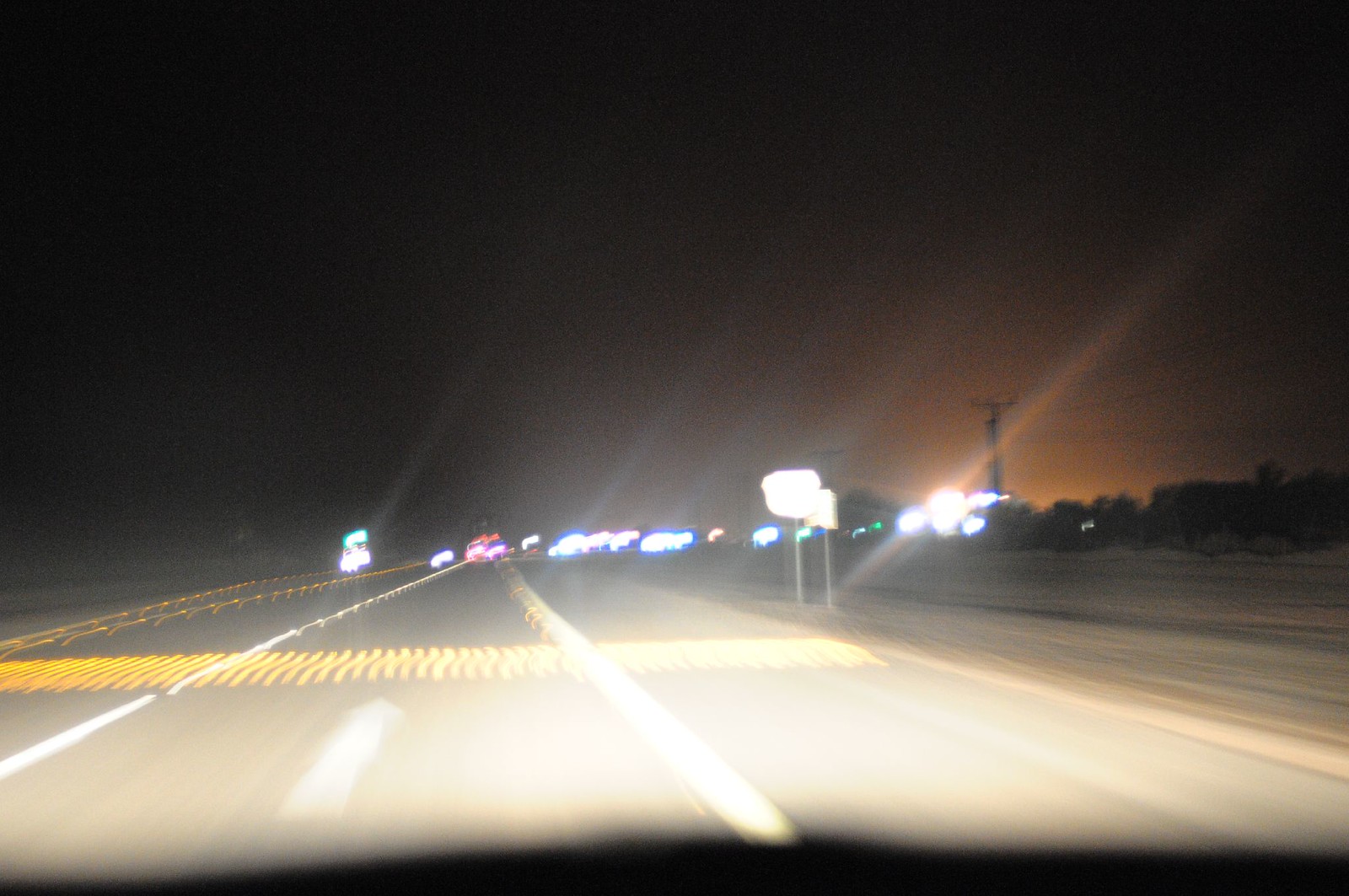This photograph, taken at night from within a car, captures the view through the front windshield. The dark asphalt highway stretches ahead, illuminated by the car's headlights. Directly in front of the vehicle, there is a yellow line of speed bumps that crosses both lanes of traffic. In the distance, the glimmer of cars' headlights dot the road, leading towards a cluster of brightly lit buildings and businesses. On the left side of the road, a well-illuminated gas station stands out against the night. To the right, a white street sign is partially visible, although its details are indistinguishable. Beyond the road on the right, an open expanse of grass extends into the darkness. The composition reflects a quiet yet vivid scene of a night drive, framed by the quiet hum of distant activity and the promise of more to come.